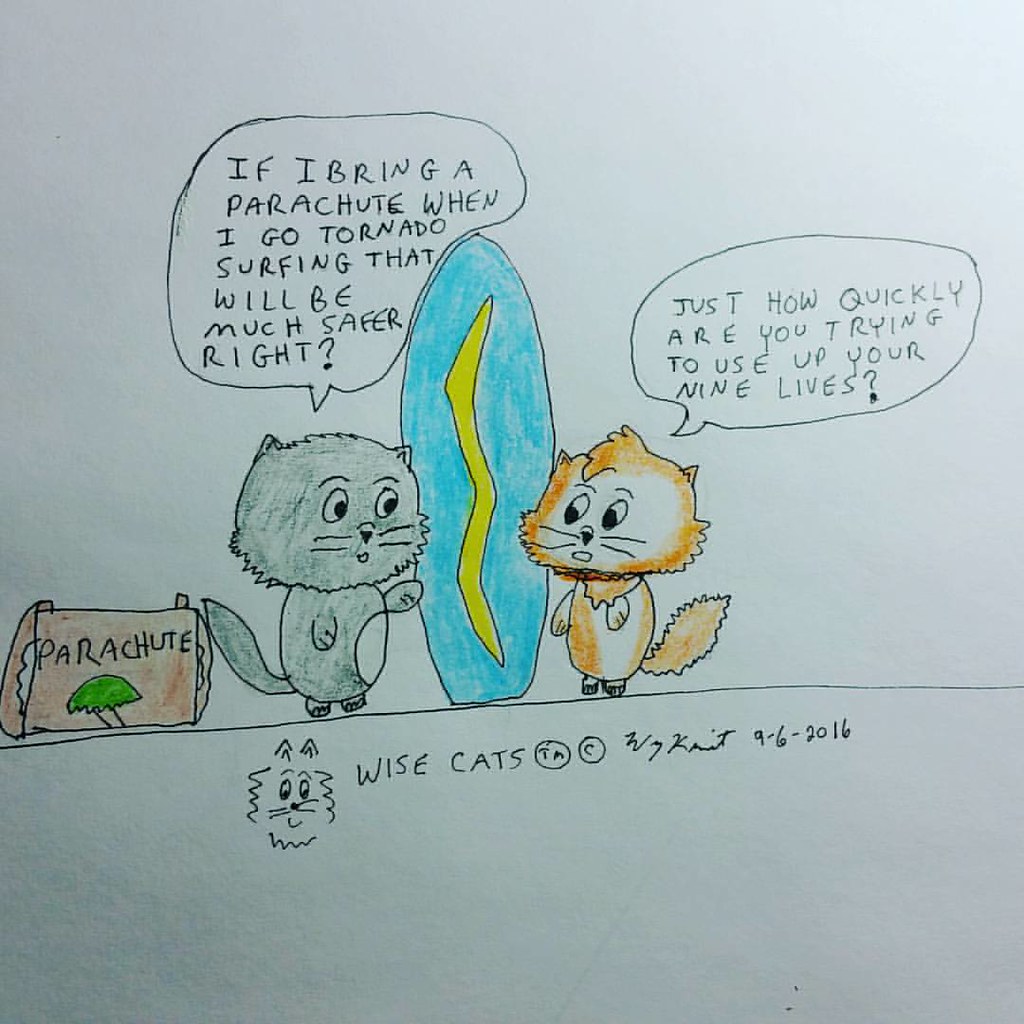This cartoon drawing features two anthropomorphic cats engaged in a humorous exchange. The cat on the left is gray and holds one paw upwards towards the item between them, a blue surfboard marked with a yellow lightning bolt pattern. To the left of the gray cat, there is a package labeled "parachute." The gray cat is quoted in a speech bubble saying, "If I bring a parachute when I go tornado surfing, that will be much safer, right?" To the right is an orange tabby cat with a white face and body patches, who responds with a concerned expression, "Just how quickly are you trying to use up your nine lives?" At the bottom of the image, there is a small drawing of a cat face accompanied by the text "Wisecats TM" and the artist's signature with the date 9-6-2016. The overall style is rudimentary, consistent with a comic strip.